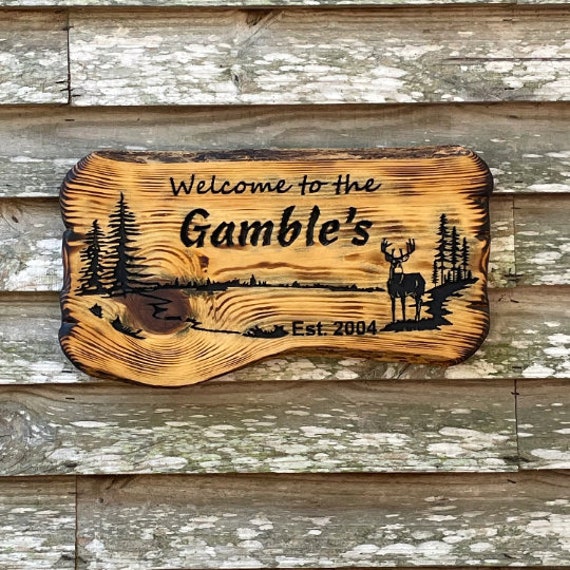The image depicts a wooden sign centered on the side of a deteriorating clapboard house or building. The building's weathered wooden boards, with peeling paint mostly gone, form the backdrop for the sign. The sign, crafted from a darker pine-colored wood, features wood-burned imagery that includes a deer and evergreen trees. These decorative elements flank the bold, capitalized text "WELCOME TO THE GAMBLES" at the top, while "Established 2004" is engraved at the bottom right. The edges of the sign appear intentionally burnt, adding a rustic charm to its overall appearance. The colors primarily include shades of pine, black, gray, and white.